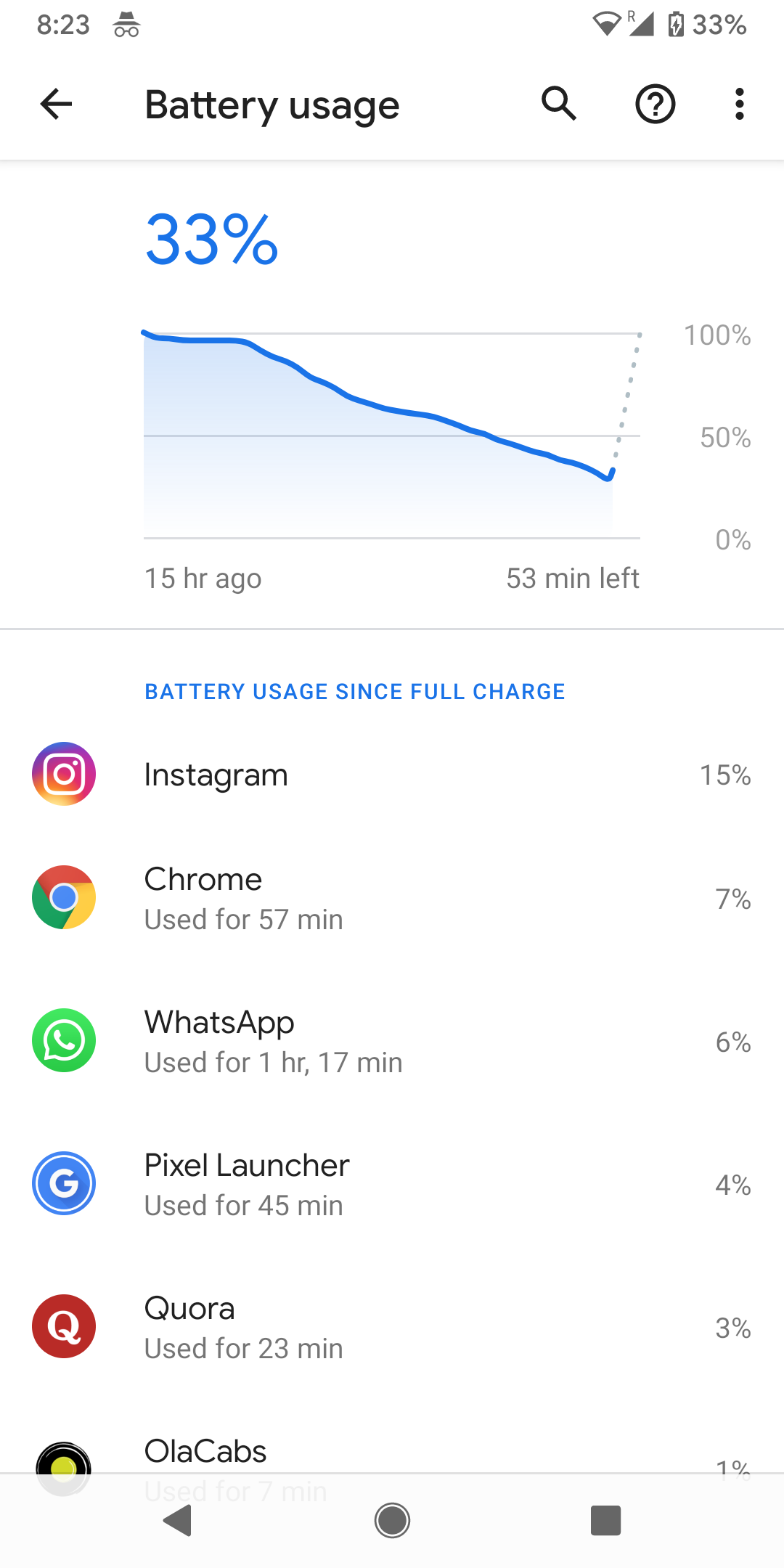The image is a screenshot taken from a smartphone, displaying detailed battery usage statistics. In the upper portion, the battery percentage is at 33%, and the current time displayed is 8:23. The user interface also shows a Wi-Fi signal icon, a triangle, and an avatar of a person with glasses and a hat.

The center section of the screenshot features a line graph depicting the battery level over time. The x-axis of the graph is labeled with time intervals, starting from "15 hours ago" on the left end and leading to "53 minutes left" on the right end. The y-axis ranges from 0% at the bottom to 100% at the top. The graph shows a declining blue line indicating the battery drain, with a dotted line suggesting the estimated time to recharge back to 100%.

The lower section of the screen details the "Battery usage since full charge" with a list of applications and their respective battery consumption percentages: Instagram at 15%, Chrome at 7%, WhatsApp at 6%, Pixel Launcher at 4%, Cura at 3%, and Ola Cabs at 1%.